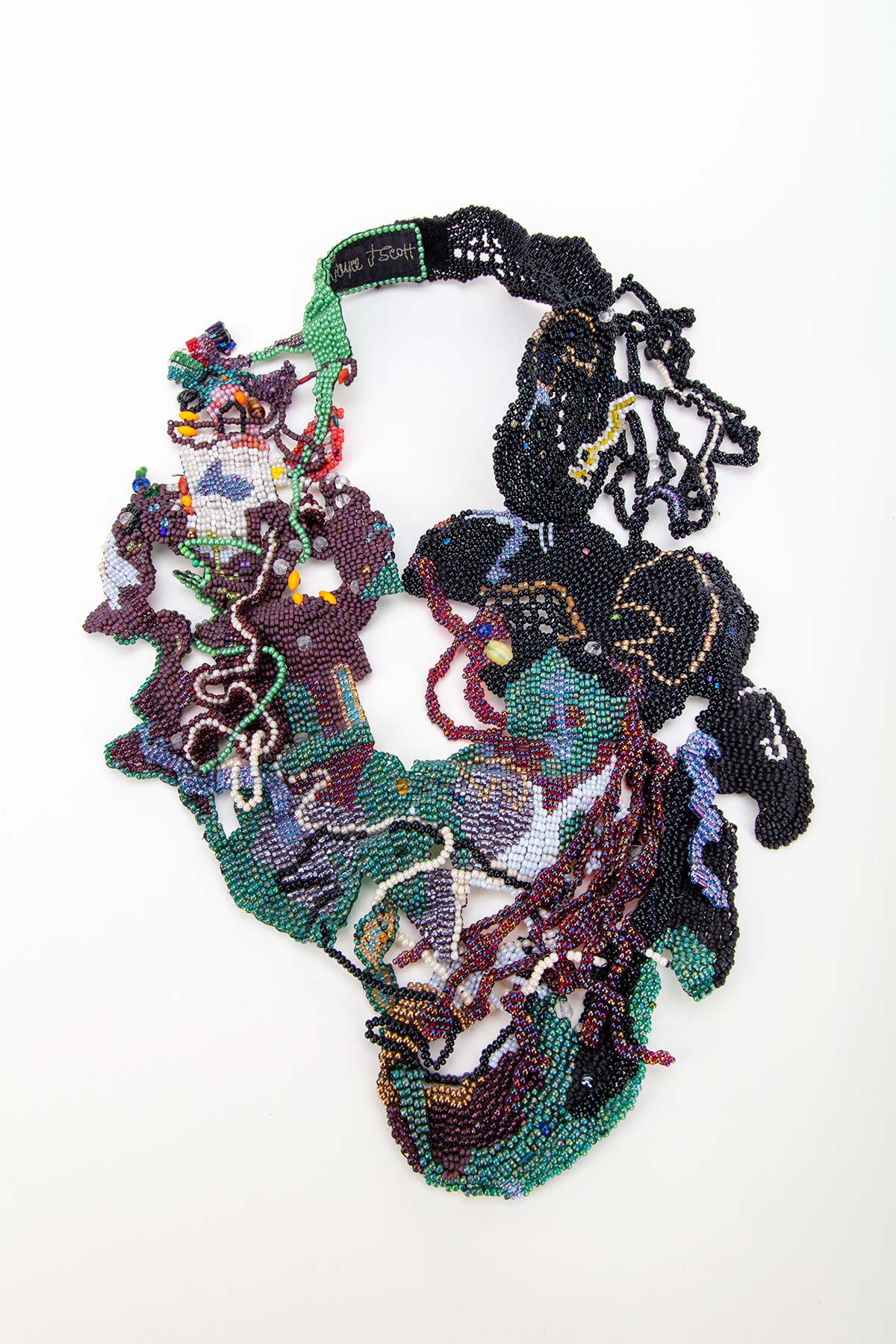The image showcases an intricate and colorful beaded item of apparel, potentially a beaded collar or scarf. The brand name "Voyage J. Scott" is partially visible on a curved label within the piece. The elaborate design predominantly consists of tiny, seed-like beads woven into a detailed pattern. At the bottom of the item, there are gray-colored beads, transitioning to blues in the middle, creating an opening that suggests it can be worn around the neck. 

The left side features intricate designs resembling windmills and flags, with curving, swirling white beads, while the right side incorporates darker hues, including deep maroon and blue beads. The overall pattern is dynamic and somewhat abstract, with various colors interwoven, such as greens, purples, whites, and reds. The item is fastened with Velcro straps at the top, allowing for easy wearability. Additional strings of beads lying on the item suggest ongoing embellishments, making it a unique and evolving piece of wearable art. This beaded creation is an exquisite example of craftsmanship, blending artistic design with functional fashion.